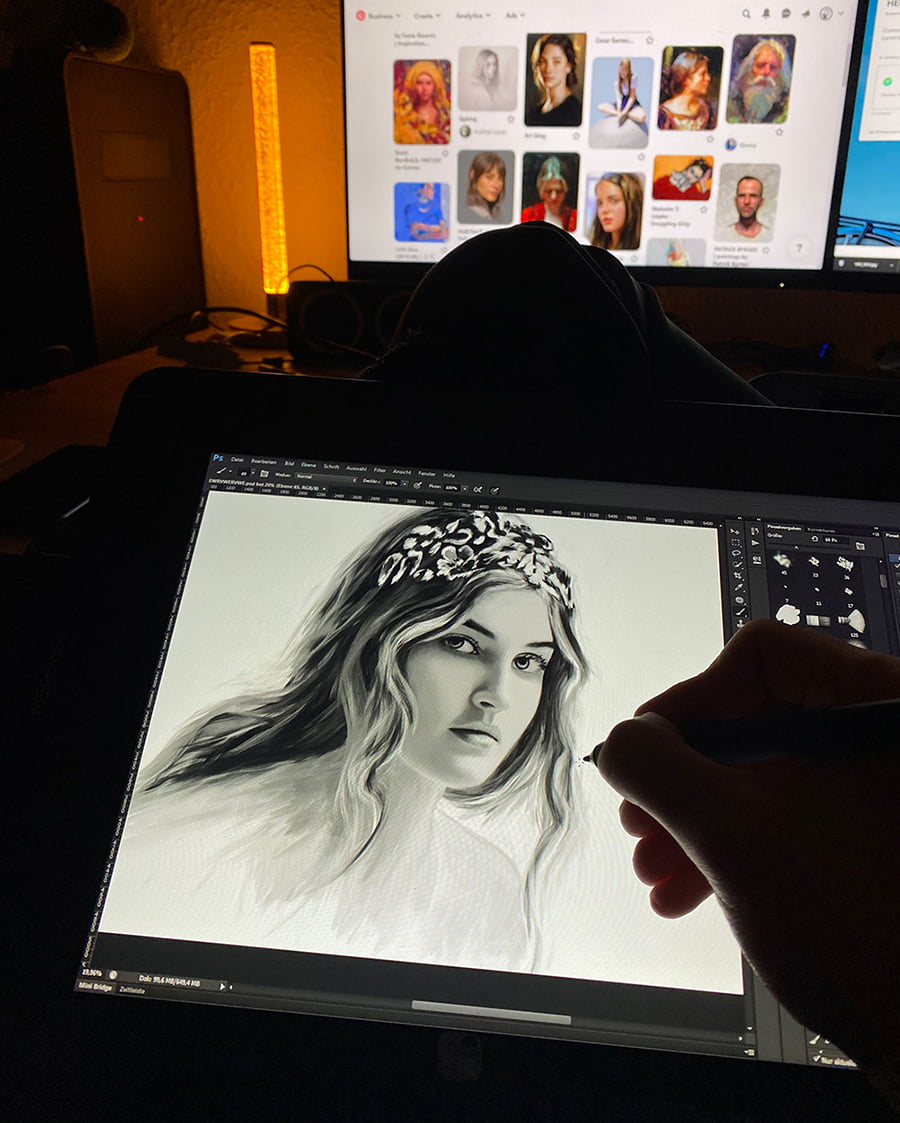In this image, a young Caucasian woman with dirty blonde or light brown hair is seen intently drawing on an electronic pad, possibly a laptop or tablet, using a stylus. She is wearing a white top and has her gaze directed off to the side. The scene is dimly lit, with the edges of the image appearing rather dark. 

In the background, the corner of a wall is visible, painted a vibrant orange, accentuated by a yellow strobe light positioned to the left. In the foreground, there is a black-rimmed white screen displaying a grid of twelve photographs against a white background. The photographs seem to be organized into two rows of six. Most of the photographs feature images of Caucasian females, with two notable exceptions: one male with a white beard positioned at the end of the top row, and another clean-shaven male with short hair located at the bottom right.

Additionally, on the bottom row, the second image from the right stands out with a cartoon-like appearance. To the right of this main screen, a smaller blue screen is partially visible, featuring a small white square. The overall composition of the scene evokes a workspace or creative studio environment.